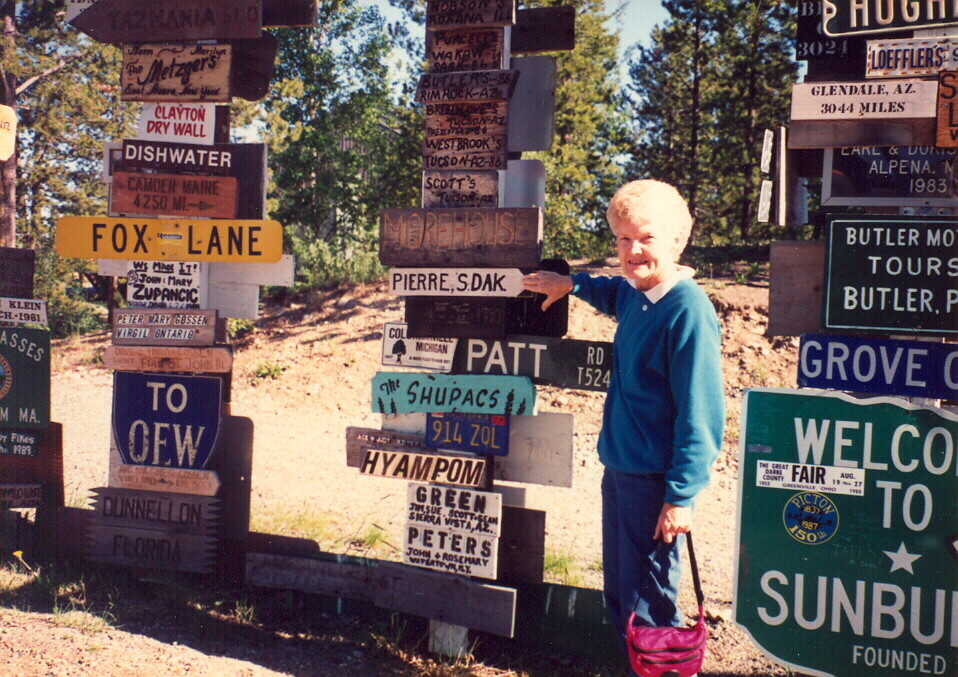In this photo, an elderly woman with short, curly white hair, dressed in a blue sweatshirt with a white collar and denim jeans, is standing in an outdoor, wooded park area with a dirt-covered hill and trees in the background. She is holding a bright pink purse with a black handle and is positioned next to one of four tall poles covered in a variety of colorful, weathered signs indicating different locations. Her hand touches a weathered white sign that reads "Pierre, South Dakota." Other signs, in various colors, fonts, and sizes, include "Fox Lane," "Dishwater," "Metzger's," "Morehouse," "The Shoe Packs," and "Camden, Maine." Some signs are metal and rusty, indicating they have been there for a long time, while others are made of wood and appear hand-carved. The scene reflects a charming mix of aged and diverse place markers, creating a nostalgic ambiance.